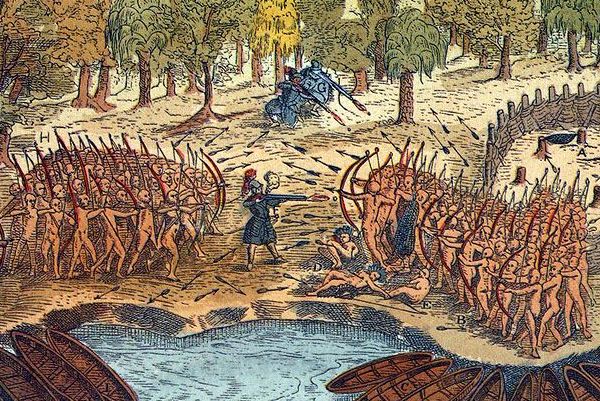The image is a vibrant, hand-drawn cartoon scene depicting a chaotic battle. At the bottom, there is a small pond or river with brown canoes piled up along both banks—approximately eight or nine canoes on the right and three or four on the left. Just beyond these canoes, large groups of naked, orange-colored indigenous or tribal people are positioned on either side of the water, about 100 on each side. They are armed with bows and arrows, facing each other and actively shooting across the scene.

Amidst the tribal conflict, a colonial settler dressed in a long coat and helmet, armed with a rifle, stands in the center, targeting the tribe on the right. Surrounding the central settler are additional figures, some crouched and shooting arrows or rifles, engaged in the intense battle.

The background features cartoonish trees with multicolored green and yellow foliage and palm-like trunks, enhancing the drawing's vivid and dynamic atmosphere. The scene is well-lit and brightly colored, capturing the intensity and drama of this tribal clash.